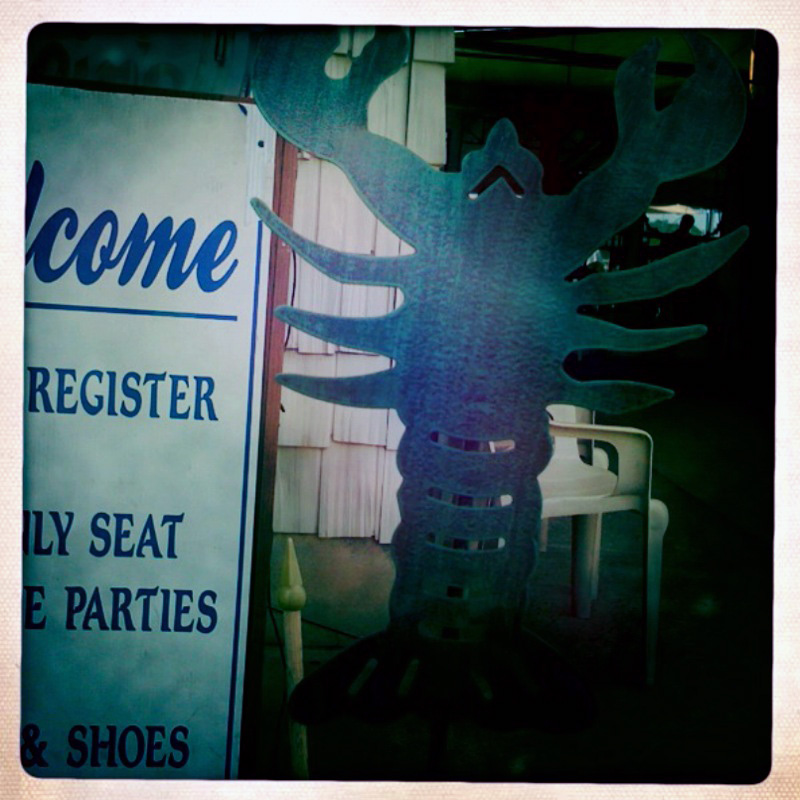The image depicts a detailed and intriguing scene centered around a unique sign display. On the right, the prominent feature is a dark gray to black metal lobster standing upright, balanced on its tail with its pincers raised in an assertive gesture. The lobster has three legs protruding from each side of its body, and the claws on its pincers are noticeably open. Behind the lobster is a white plastic chair, emphasizing the lobster's metallic texture and intricate design.

To the left of the lobster, a white signage board with blue text partially obscured comes into view, featuring words like "welcome," "register," "seat," "parties," and "choose." The implication is a welcoming message, possibly for a restaurant or a similar establishment. Both the metal lobster and the sign are mounted on poles or stands, contributing to the organized display.

In the background, the exterior wall of a building is visible, hinting at the establishment's structure. An interior section can be seen where a person is seated, and additional white or cream chairs are arranged, creating an inviting atmosphere. The upper right part of the image shows a darker area with a silhouette, adding depth and context to the overall scene.